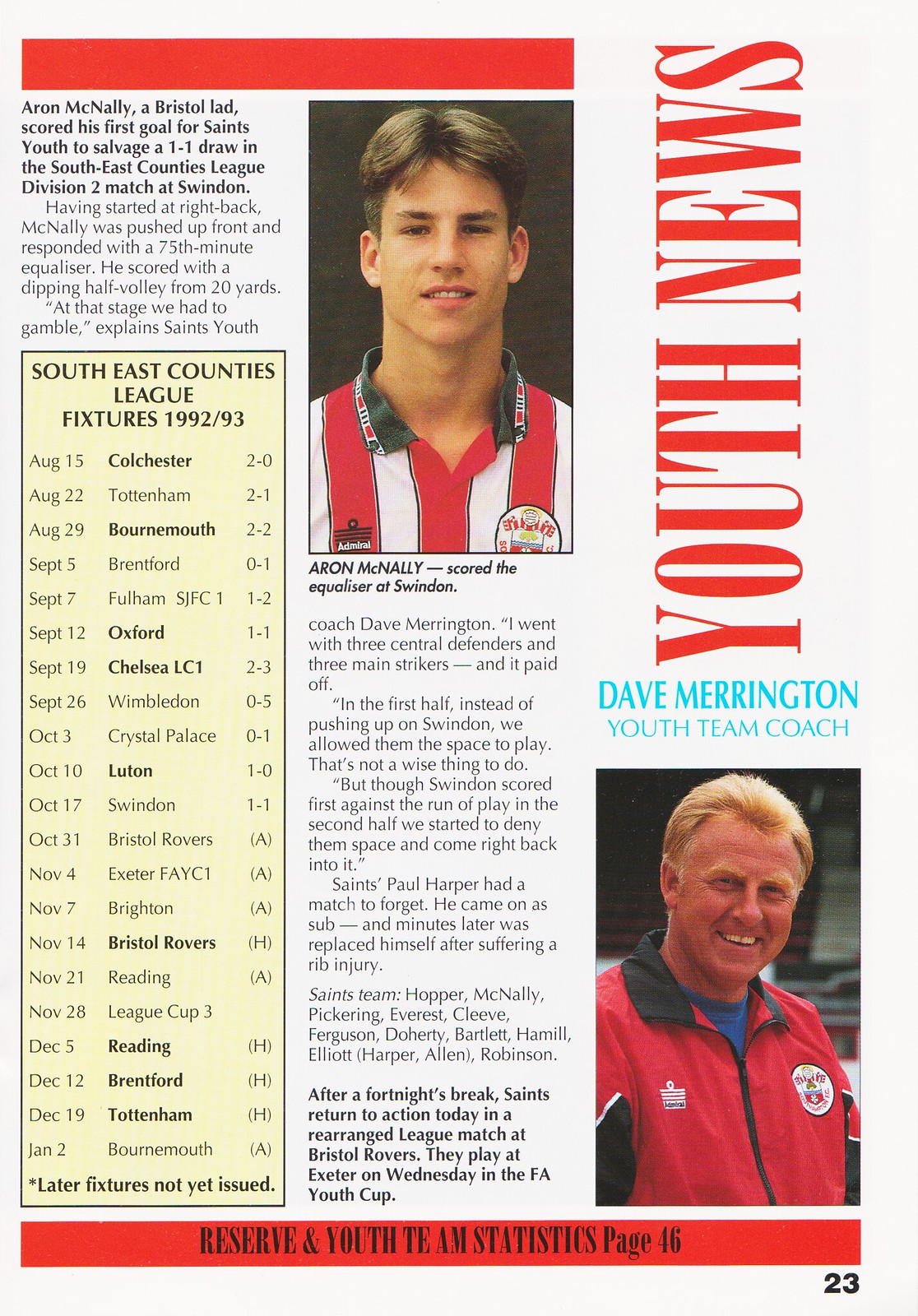The image is a detailed page from a magazine titled "Youth News" oriented vertically in bold red text on the top right. The page features an article about Aaron McNally, a young footballer. In the upper left, a horizontal red stripe stretches two-thirds across the page. Below the stripe, centrally positioned, is a picture of Aaron McNally, a Caucasian young man with short brown hair parted slightly to the left of the center. He wears a red and white vertically striped shirt displaying a white symbol on the upper right chest. Underneath his image, a caption reads: "Aaron McNally scored the equalizer for Swindon." 

The article details how McNally, who started as a right back, was moved upfront during a match against Swindon, where he scored a pivotal 75th-minute equalizer with a dipping half volley from 20 yards. A quote from the coach, Dave Merrington, highlights the tactical gamble taken by the team. Portions of the article describe how the team initially allowed Swindon space, leading to Swindon’s first goal, but constrained them in the second half to make a comeback.

Below the article, in bold print, an update indicates the team's next matches after a fortnight's break, starting with a league match at Bristol Royals and a fixture at Exeter in the FA Youth Club Cup. To the right of McNally's picture, there is an image of Coach Dave Merrington, a Caucasian man with short blonde hair, wearing a black jacket with distinct white symbols. Above his photo, in blue text, it says "Dave Merrington, Youth Team Coach."

The background of the page is predominantly white, formatted in portrait orientation, taller than wide. In the lower right corner of the page, in black print, is the number 23. On the left, a rectangular column with a yellow background lists Southeast Counties League fixtures for the 1992-93 season, player names, match locations, and corresponding scores. Additionally, toward the bottom, it notes "Reserve and Youth Team Statistics" on page 46.